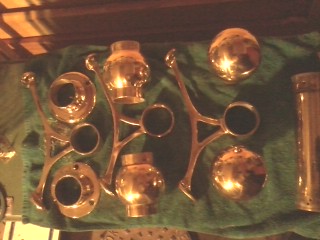This photograph captures a small, detailed arrangement of brass-colored and chrome-colored fittings, likely components for a banister rail. The setting appears to be on a green terrycloth towel, with a light wooden surface and sunlight casting shadows in the background. The image includes several shiny brass fittings arranged horizontally. On the left, there are multiple tiers of brown and orange hued sections transitioning into yellow and dark brown stripes and patterns. Centrally placed are fittings with a brassy color, featuring circular openings designed to hold a wooden rail. These fittings are connected by brassy globes and balls; the middle piece particularly stands out with brass spheres between two segments. On the far right is a long, bronze tube with holes at the ends for wooden inserts. The overall impression is a close-up view of intricate, possibly handmade, banister components, each precisely designed for assembly with wood to form a stair railing.